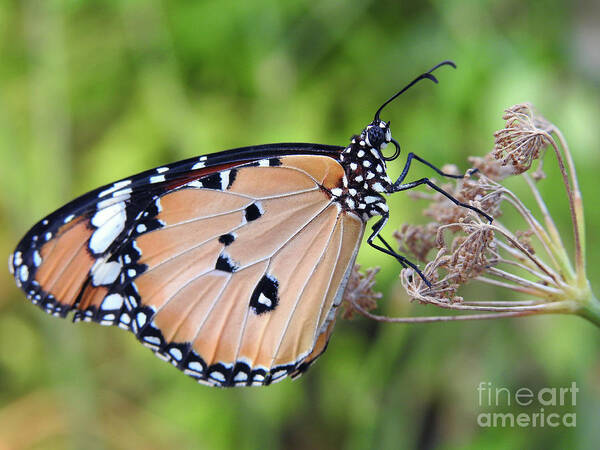This outdoor, close-up color photograph captures a beautiful monarch butterfly as the central focus. The butterfly, perched delicately on a peculiar brown plant with tiny spheres and a green stem, displays its striking orange wings edged with black and decorated with white dots. Its black body also features prominent white spots, complemented by long black legs and antennae. The background is a lush blur of green foliage, suggesting an abundant, vibrant natural setting. At the bottom right, the image is discreetly watermarked with "Fine Art America."